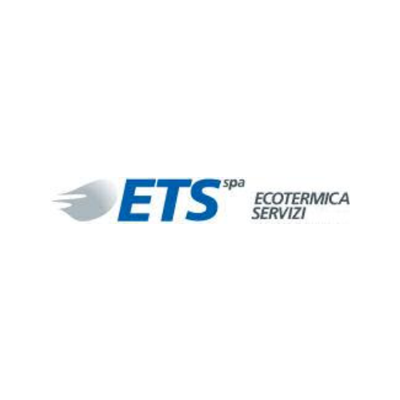The image features a company logo centered against a solid white background, taking up about 10% of the space. Dominating the logo is the prominently bold, all-caps dark blue text "ETS," followed by a smaller "SPA" in gray located in the upper right-hand corner of the "S." To the left of "ETS," there's a rounded, gray, swoosh-like pattern with streaks extending outward, evoking a sense of motion. Directly to the right of "ETS SPA" is the dark gray text "ECOTERMICA" in uppercase, beneath which is "SERVIZI." The overall impression is that of a contemporary business logo, utilizing a minimalist color palette of white, dark blue, and gray. The composition and design elements suggest this logo might be used on company stationery or branding materials.